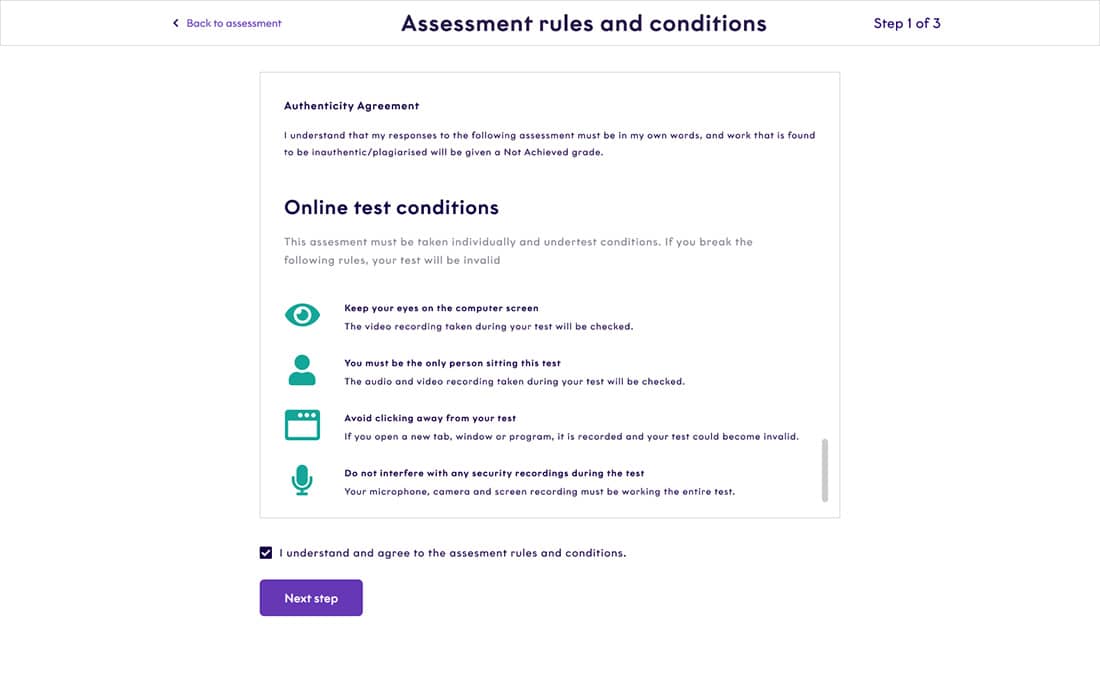This screenshot features a webpage displayed on a desktop monitor in landscape orientation, with a white background and predominantly black, gray, and purple text. At the top of the screen is an outlined title bar. Centrally positioned in black text, it reads "Assessment Rules and Conditions." On the left-hand side, a purple text labeled "Back to Assessment" accompanies a left-pointing arrow. To the right, it indicates "Step One of Three."

Beneath this section, a gray outlined box contains the heading "Authenticity Agreement." This section emphasizes, "I understand that my responses to the following assessment must be in my own words, and work that is found to be inauthentic/plagiarized will receive a not achieved grade."

Further down, under the subheading "Online Test Conditions" in black text, a gray text block states, "This assessment must be taken individually and under test conditions. If you break the following rules, your test will be invalid." Following this are four specific rules, each accompanied by a corresponding teal-colored icon to the left.

1. The first rule, illustrated by an eye icon, mandates, "Keep your eyes on the computer screen. The video recording taken during your test will be checked."
2. The second rule, paired with a user icon, instructs, "You must be the only person sitting this test. The audio and video recording taken during your test will be checked."
3. The third rule states, "Avoid clicking away from your test."
4. The final rule warns, "Do not interfere with any security recordings during the test."

Each rule is clearly designed to ensure the integrity and security of the online assessment process.